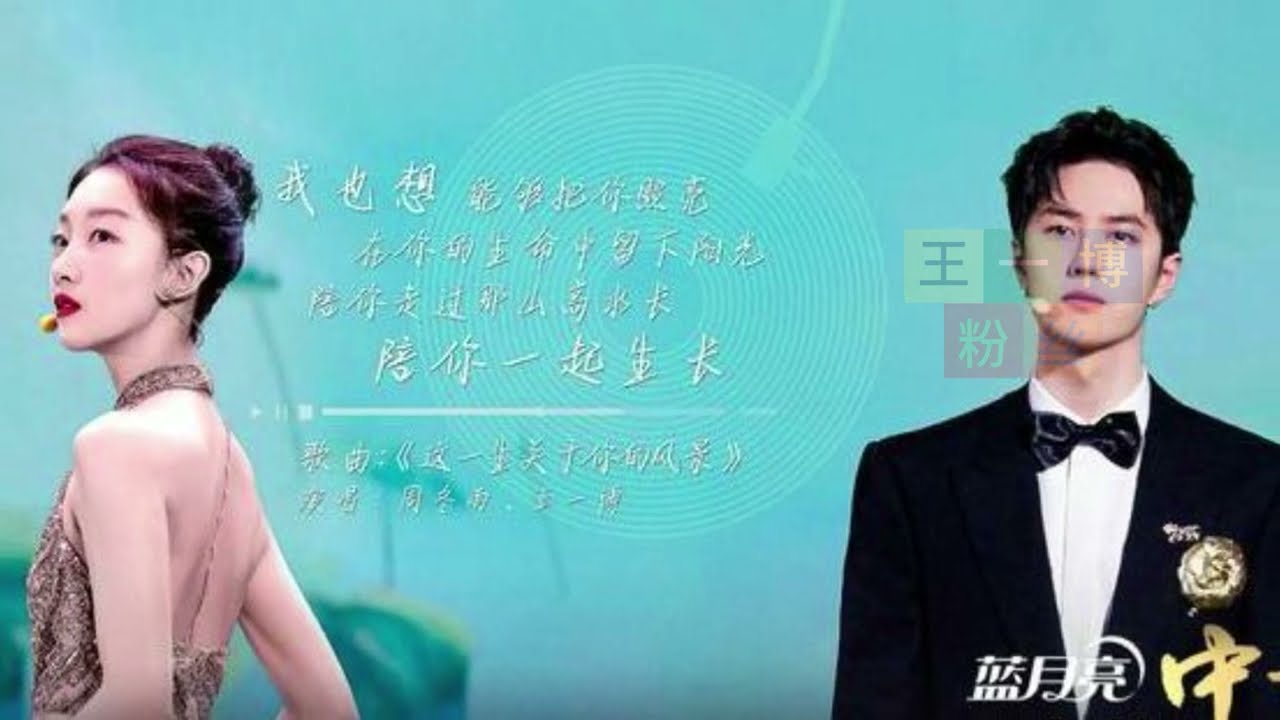The image features a potential advertisement with text in an East Asian language, suggesting it might be Japanese or Chinese. The background is mainly light blue or turquoise, decorated with both white text and perhaps 20 concentric light green circles in the center. 

On the left side of the image, there's a young Asian woman with fair skin, captured in a profile view as she looks over her left shoulder. She is adorned in a fancy, sleeveless, and backless gold dress that wraps around her neck with a thin strap. Her hair is styled in an elegant bun, and she wears bright red lipstick. Close to her mouth, there's a small yellow microphone, with a wire extending from her ear, hinting at her role as a singer.

On the right side, there's a young Asian man with fair skin as well. He is dressed in a stylish black tuxedo, featuring a black bow tie with gray swirls, and a white shirt. His dark, thick hair complements his formal look. Additionally, there is a medallion-like accessory on the left side of his chest. Both individuals are likely in their late teens or early twenties, and their poised expressions further emphasize the formal and possibly celebratory nature of the scene. The lower right corner of the image also contains more white text in the foreign language.